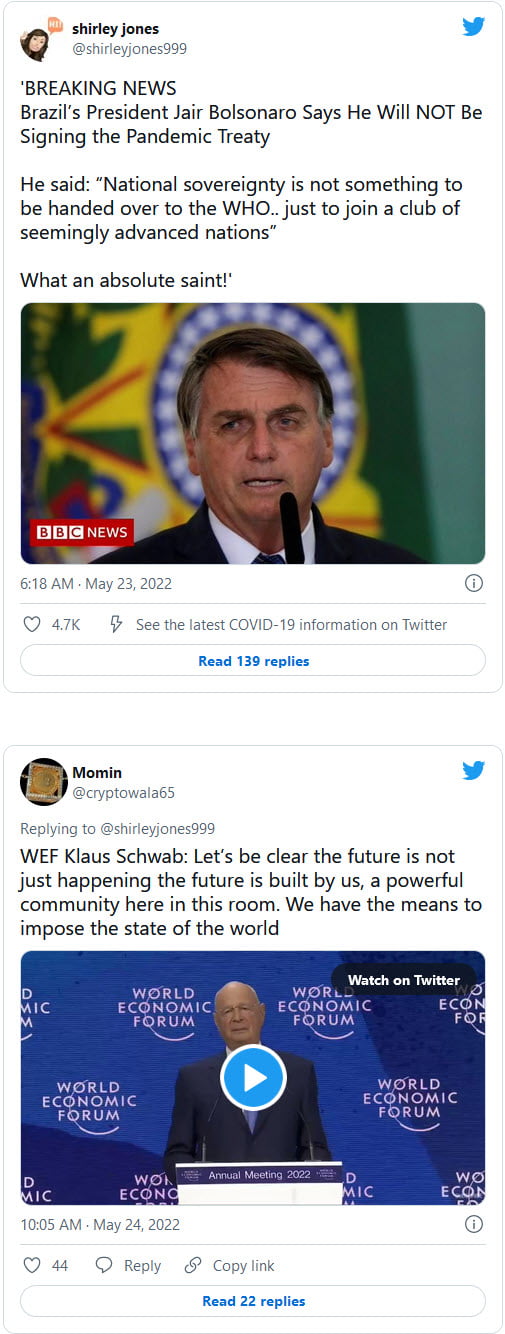The image displays a couple of posts on the social media platform X (formerly known as Twitter). The user interface includes a picture of the old Twitter Blue Bird logo in the upper right-hand corner.

The top post features an icon of a woman's face in the upper left corner, belonging to the user Shirley Jones (@ShirleyJones999). The post includes the headline: "Breaking News! Brazil's President Jair Bolsonaro says he will not be signing the pandemic treaty. He stated that national sovereignty is not something to be handed over to the WHO, just to join a club of civically advanced nations. What an absolute saint!" 

This post is accompanied by a photograph showing a man in a suit, standing in front of a microphone, with the bottom corner labeled "BBC News." Below the image, the timestamp reads "6:18 AM, May 23, 2022," followed by a reminder to "See the latest COVID-19 information on Twitter." The post has generated 139 replies.

The second post is a reply from the user Momen (@CryptoWalla65), responding to Shirley Jones. This post quotes WEF Chair Klaus Schwab: "Let’s be clear, the future is not just happening. The future is built by us, a powerful community here in this room. We have the means to impose the state of the world." This message is paired with a video still, featuring an older man at the World Economic Forum, standing at a podium with a backdrop that reads "World Economic Forum." There's a play button superimposed over the video. Below this video, the timestamp reads "10:05 AM, May 24, 2022," and the post has 22 replies.